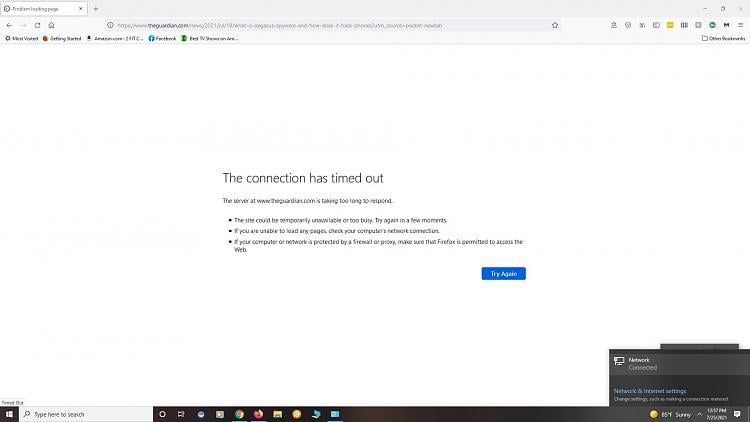A blurry and faint screenshot of a computer monitor displaying a web browser page. At the top of the browser, a light gray bar is visible with a search bar in the left upper corner containing some illegible black text, possibly including the words "landing page." On the right side of the bar, there are three black icons—a minus sign for minimize, a square for maximizing, and an X for closing the window.

Below this bar, the left side of the toolbar features a gray back arrow, a forward arrow, a reload symbol, and a home button. In the center of the toolbar, the URL field displays "theguardian.com" followed by a lengthy URL. To the right of this field, there's a star icon for bookmarking the page. In the upper right corner of the toolbar, there is a horizontal line of icons that are too blurry to be identified clearly.

The bookmarks toolbar underneath this section on the left edge lists several bookmarks: "most visited," "getting started," an illegible entry, "Facebook" marked by its blue icon, and another entry with a green icon.

The main content area of the webpage against a white background shows an error message: "The connection is timed out. The server at www.theguardian.com is taking too long to respond." To the left of this message, three black bullet points suggest troubleshooting steps such as checking your connection and ensuring the firewall isn't blocking the site. At the bottom right corner of this section, a blue rectangular button with white text reads "Try again."

At the very bottom of the image, the black Windows taskbar is visible. It features the black Windows logo on the left, a search bar to its right, and a series of frequently used program icons further to the right. In the bottom right corner, a gray pop-up window indicates "Network connected" in white text.